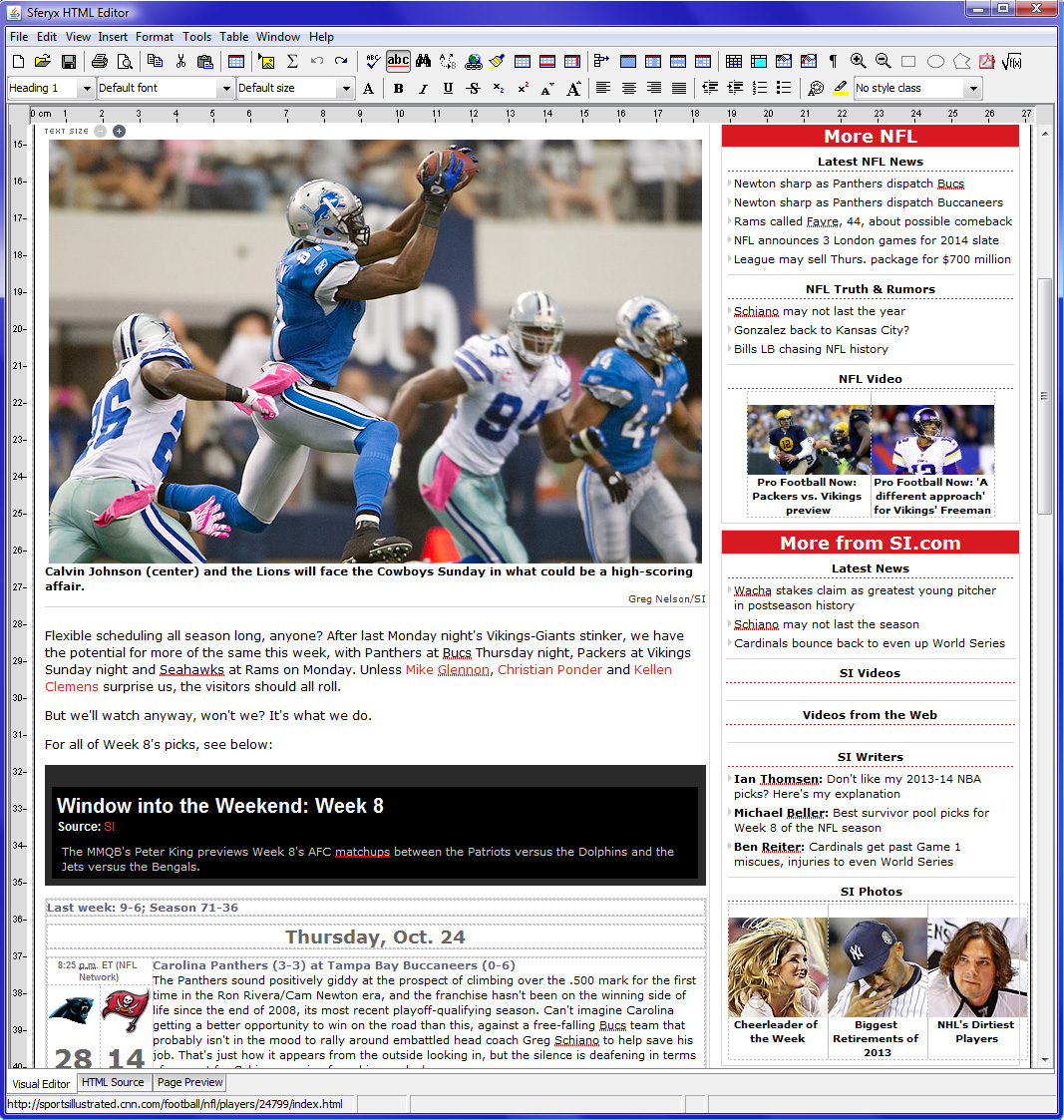The image displays a web browser window open on a desktop computer, identifiable by the icons for minimize, maximize, and close located at the top right corner. The top left corner labels the application as "Spherix HTML Editor," accompanied by a Java icon. The editor's interface includes a menu bar at the top with tabs such as File, Edit, View, Insert, Format, Tools, Table, Window, and Help.

The right side of the editor features a scrollbar and additional editing options. At the center of the screen, there is a picture of football players on the field; the players in blue jerseys are facing opponents in white jerseys. Below this image, text reads: "Calvin Johnson Center, and the Lions will face the Cowboys Sunday in what could be a high-scoring affair."

Further down, the text discusses the flexibility of schedule for the season: "After last Monday night's Viking Giant Stinker, we have the potential for more of the same this week with Panthers at Bucks Thursday, Mad Packers at Vikings Sunday night, and Seahawks at Rams on Monday unless Mike Glenn, Christian Pond, and Kellen Krems surprise us. The visitors should all roll." The names in this section are highlighted in red.

On the left side of the editor, a navigation pane lists various links: More NFL, Latest NFL News, NFL Truths and Rumors, NFL Video, More from SI.com, Latest News, SI Videos, Videos from the Web, SI Writers, and SI Photos.